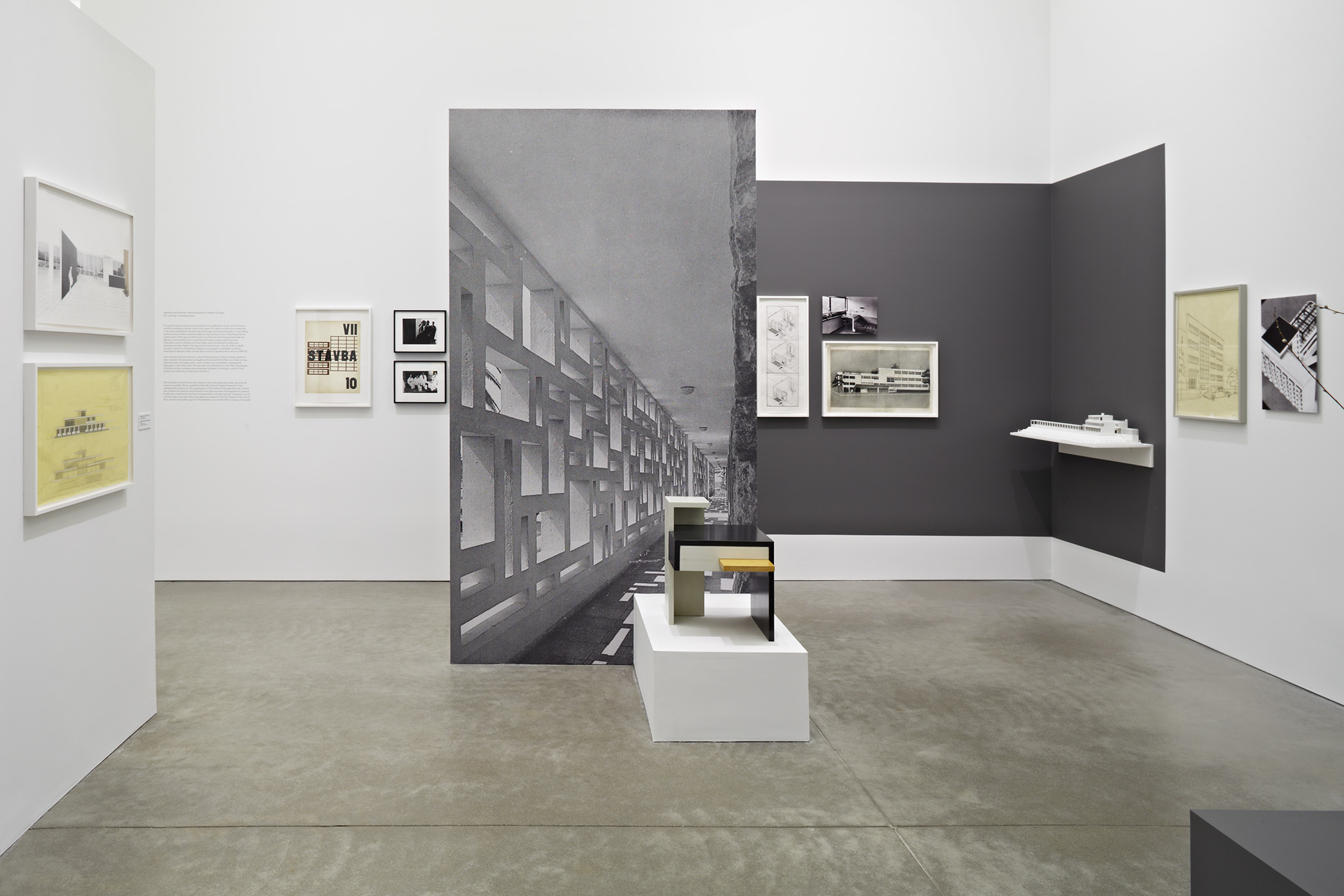This photograph captures a meticulously arranged art installation, likely within an art museum showcasing architectural design themes. The room's ambiance is defined by large grey floor tiles and pristine whitewashed walls adorned with various framed illustrations and prints.

On the left side of the room, there are two framed pictures; one exhibits black geometric shapes on a whitish background, and the other seems to have a greenish tint. Moving to the center of the room, three more framed illustrations are displayed, accompanying a large panel that appears to depict a building. Below this panel rests a white pedestal supporting a detailed 3D model, serving as the exhibit's focal point. 

The right side of the room features additional prints and design maps hung on a dark gray section of the wall. Further to the right, a large picture can be seen leaning against the wall, hinting at more artwork displayed beyond the frame. The text around the exhibits is not legible, adding a layer of mystery to the display. The room is filled with a range of colors such as dark grey, various shades of yellow, pale tones, and black, which contrast beautifully with the traditional gallery setting.